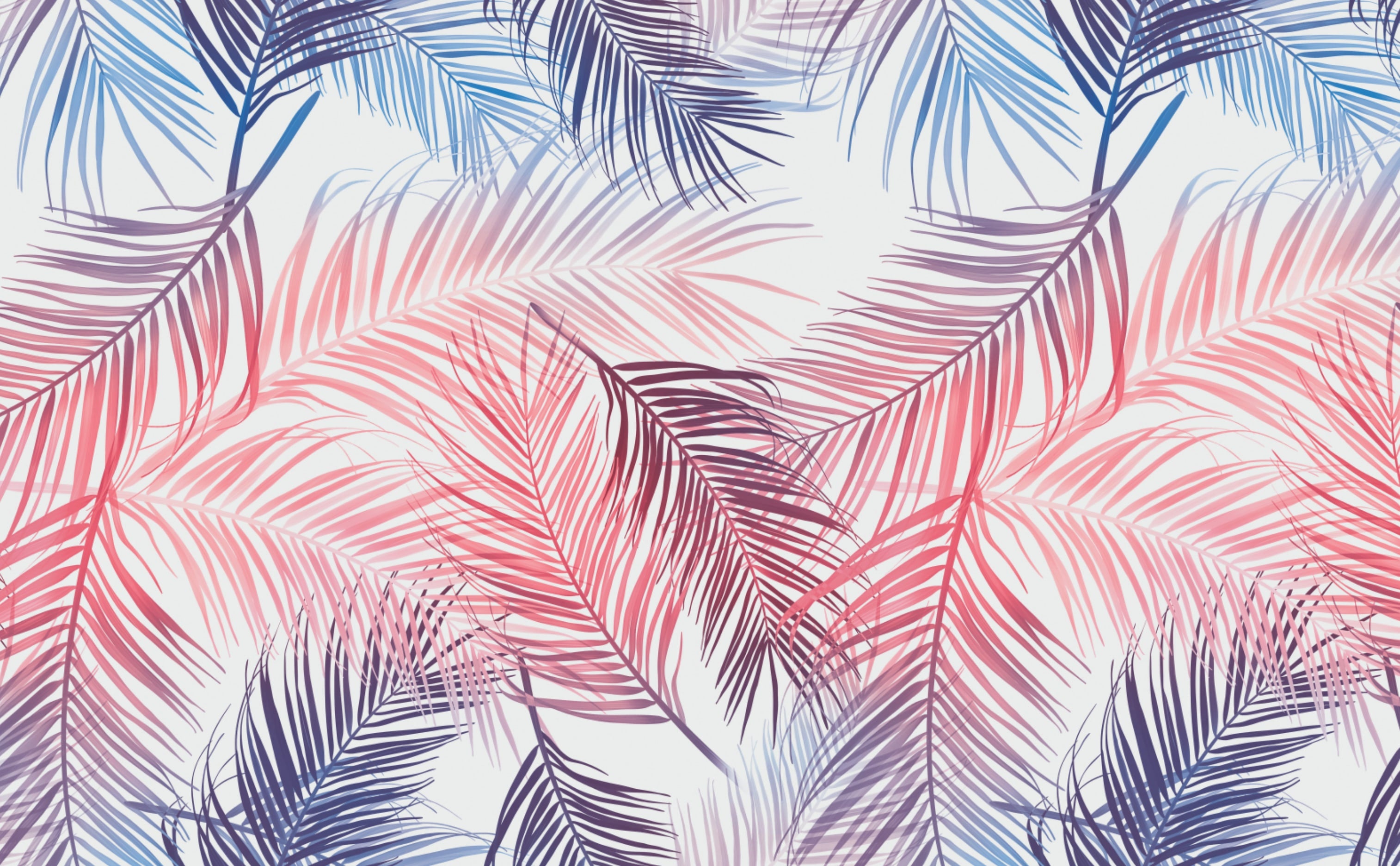This vibrant, tropical painting features a close-up pattern of multicolored palm fronds and stylized leaves against a bright white background. The foliage, in shades of blue, pink, red, and light green, is depicted with a wavy, dynamic quality, with leaves extending in numerous directions. The white backdrop shines through, creating striking silhouettes and adding a sense of depth and movement to the composition. The design captures the essence of a lush, exotic paradise, with varying densities of fronds that leave some areas densely packed while others are more sparse, enhancing the intricate and decorative nature of this stylized imagery.